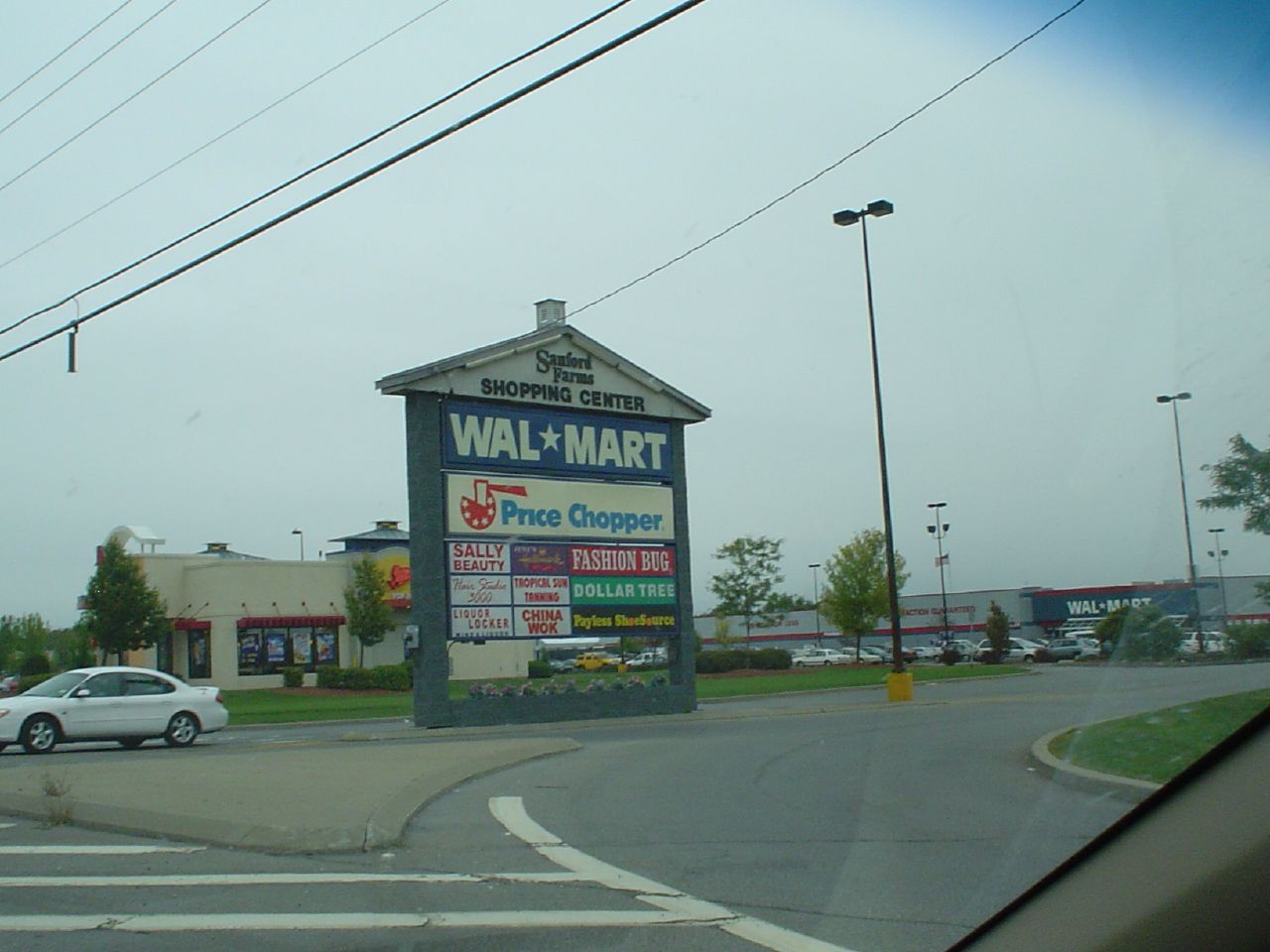The image is a vibrant color snapshot seemingly taken from a car window, possibly the side or front windshield. A narrow sliver of the car's interior frame is visible, along with some reflections and water spots on the glass. Dominating the scene are white pavement markings that resemble crosswalk stripes and a right-turn lane leading into a shopping center.

In the background, a large Walmart sign is prominent, illuminated by tall security lights and surrounded by various smaller store signs. The shopping center, identified as Sanford Farms, features a sign with a peaked roof design and fluorescent bulbs, topped with a cupola. Other stores include Price Chopper, Sally Beauty, and what appears to be Tropic Sun Tanning, along with a Dollar Tree, Liquor Locker, China Walk, and Payless Shoe Store.

To the left of the image, a white sedan, resembling a Ford Taurus, is captured mid-motion, driving from right to left. Behind it stands a low, yellow brick building with red awnings, likely a restaurant, though the name is indiscernible.

There is a wedge-shaped median of concrete separating the turning lane from the potential crosswalk area, bordered by grass curbs and a few scattered trees. Overhead, a network of utility wires crisscrosses the top left of the photo, adding an urban element to this snapshot of a bustling shopping center entrance.